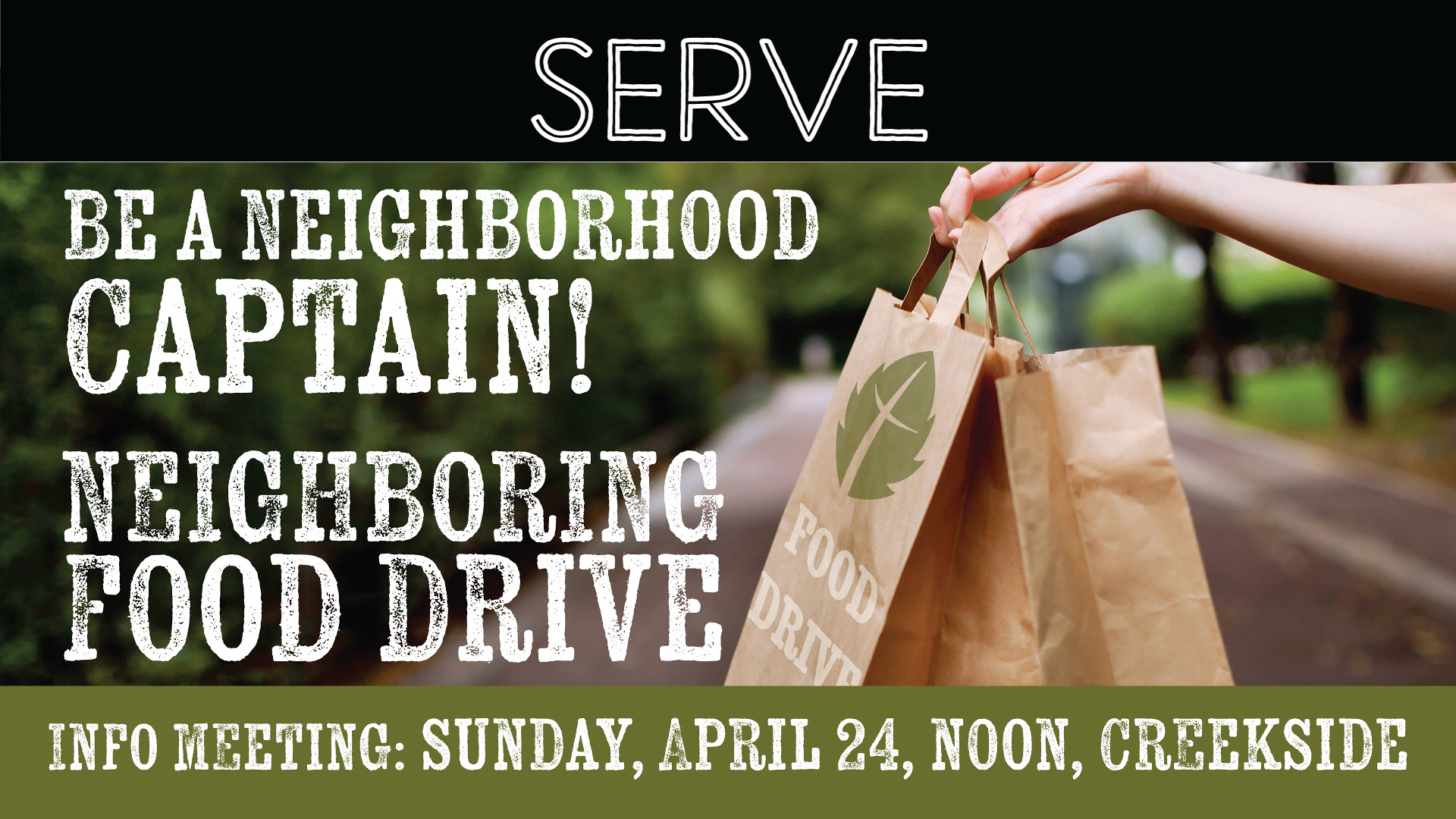This wide rectangular advertisement poster features a striking black stripe running across the top with the word "SERVE" prominently displayed in all capital letters, characterized by a thin black line within each white letter. Positioned below is a central image depicting a hand extending from the right, holding two brown paper bags adorned with a leaf design, set against a blurry background of a road and trees. To the left of the hand, the text "BE A NEIGHBORHOOD CAPTAIN!" is displayed in bold white capital letters, announcing a neighboring food drive. The bottom of the poster is bordered by a shorter olive green stripe with all capitalized white letters that provide details for an info meeting scheduled for Sunday, April 24th at noon, located at Creekside.